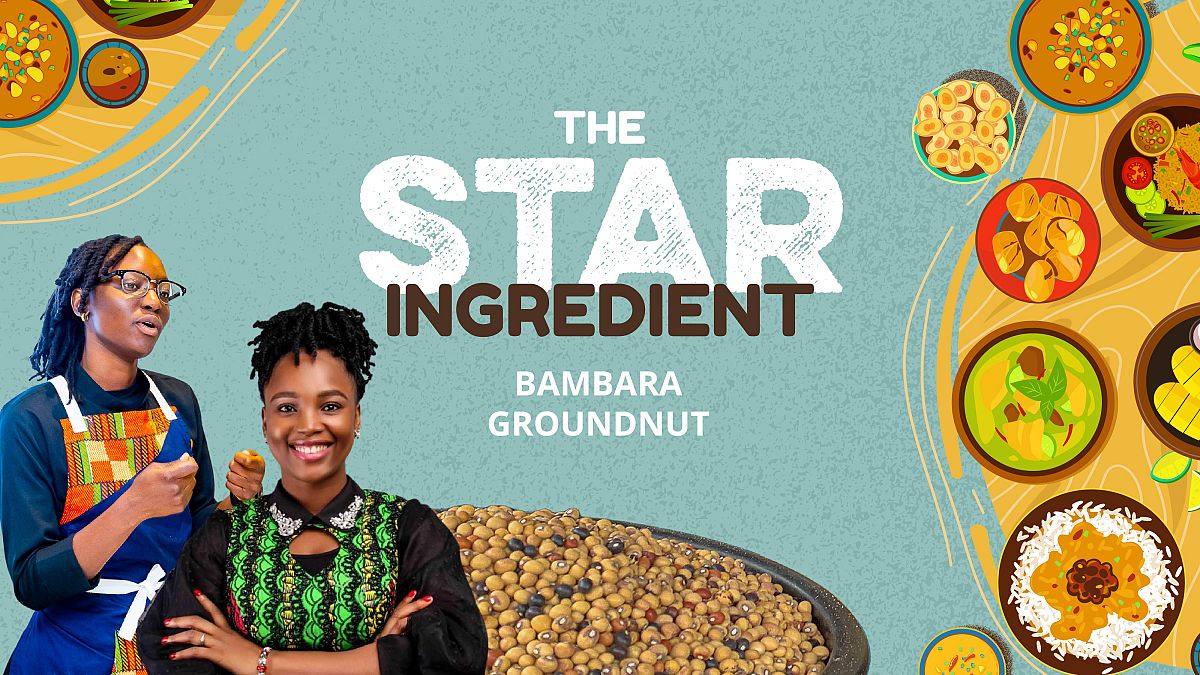Front Cover of "The Star Ingredient: Bambara Groundnut" Cookery Book / YouTube Cooking Show Thumbnail

In bold white letters, the title "The Star Ingredient" dominates the center of the image, followed by the subtitle in black letters, "Bambara Groundnut." Below this, in white letters, is the focus ingredient, "Bambara Groundnut."

The top left corner features charming cartoon-style illustrations of various food items, set against a textured brown desert backdrop with rippled edges. This desert transitions into a vast expanse of blue, suggesting a river or body of water that fills the majority of the background.

The right side of the image mirrors the desert background, filled with an enticing array of salads, bowls of nuts and seeds, and an assortment of bread, curries, and other salad-style dishes. A prominent brown dish in the bottom right corner showcases white rice topped with a vibrant yellow curry.

In the bottom left corner, two women of African descent are featured. The woman on the left, with dark brown skin, wears black glasses and her black hair is tied in a ponytail. She sports a blue top with three-quarter sleeves, revealing her forearms, and an apron with white straps and a colorful orange section adorned with green, orange, and yellow rectangles. The woman on the right, also with dark brown skin, wears a black-sleeved top with a green patterned torso section. She accessorizes with a wristband on her left arm and has pink fingernails. She smiles brightly, displaying white teeth, and her black frizzy hair is tied up. To her right is a large bowl brimming with a variety of seeds and nuts, prominently featuring the Bambara groundnut.